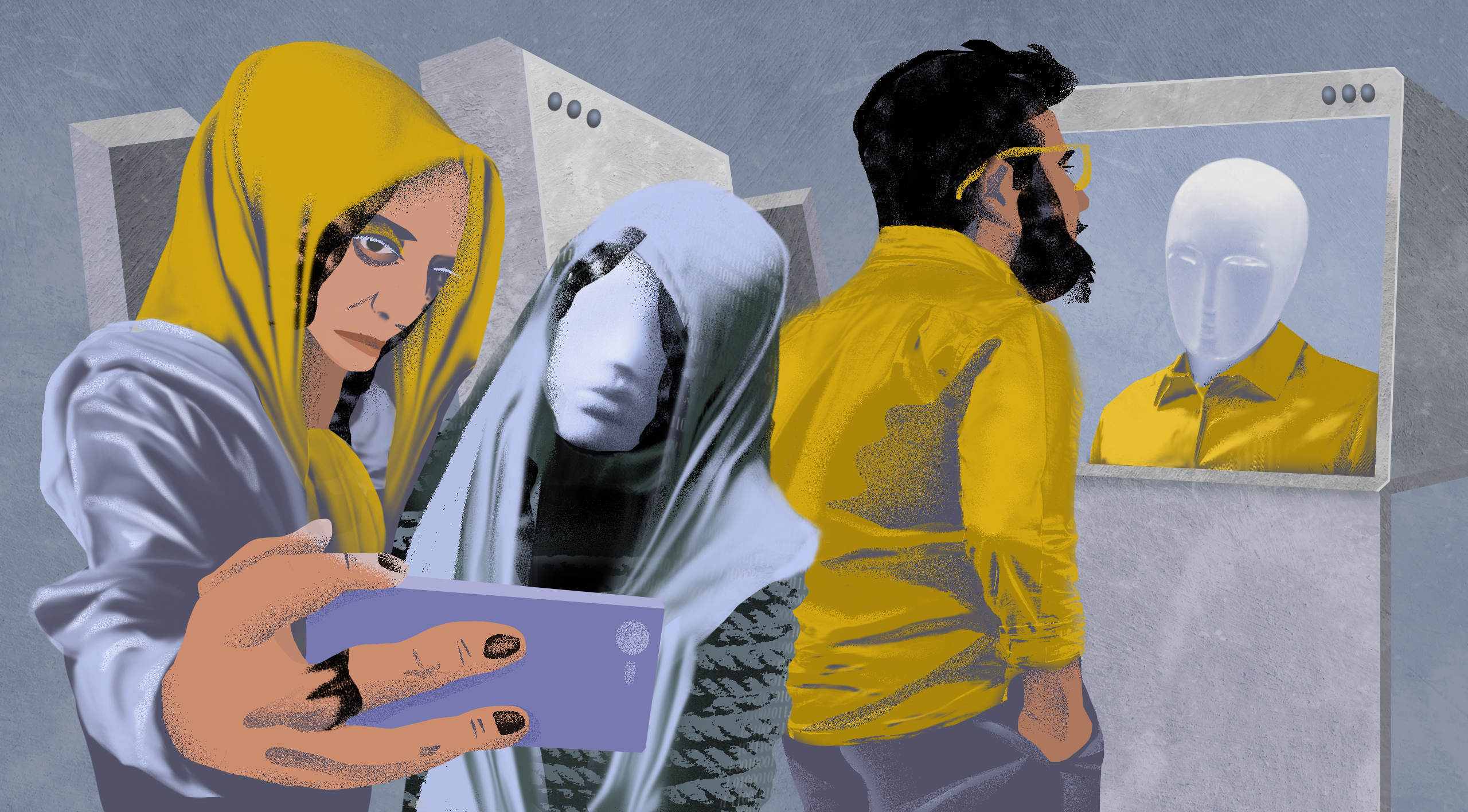The painting presents a vividly detailed scene framed by a predominantly bluish-gray atmosphere, enriched by unique individual portrayals and symbolic undertones. On the left, a woman with light brown skin, adorned with black pupils and pink lipstick, captures a selfie on her purple phone. She wears a yellow hood over her brown hair, contrasted by a gray and blue sweatshirt that becomes darker near the phone. Her hands, detailed with black painted fingernails and a small tattoo, emphasize her vibrant yellow undershirt.

To her right stands a mysterious figure, appearing as a shadowy form with a gray face, black hair, and restrained by gray ropes, donned in a gray head covering. This figure adds an element of enigma to the composition.

Central to the image is a man clad in a yellow shirt and glasses, characterized by short black hair, a long beard with sideburns, and gray pants. His hands are casually tucked into his pockets as he faces a monitor perched on a large gray square container. The monitor depicts a bald figure donning a yellow dress shirt, distinguished by a white face with blue accents around the eyes, nose, and mouth, highlighting an abstract reflection of the man himself.

Behind this central man, partially obscured, is another monitor with three dark gray circles on the left, mirroring the first. The space is defined by the gray outline of a door to their left, adding depth and separation to the scene. The two figures behind the central man also evoke curiosity as they observe the woman taking her selfie, grounding the abstract elements in a relatable human activity.

Overall, the composition integrates gray tones and yellow highlights to create a cohesive yet symbolically rich narrative, reflecting themes of self-perception and digital interaction.